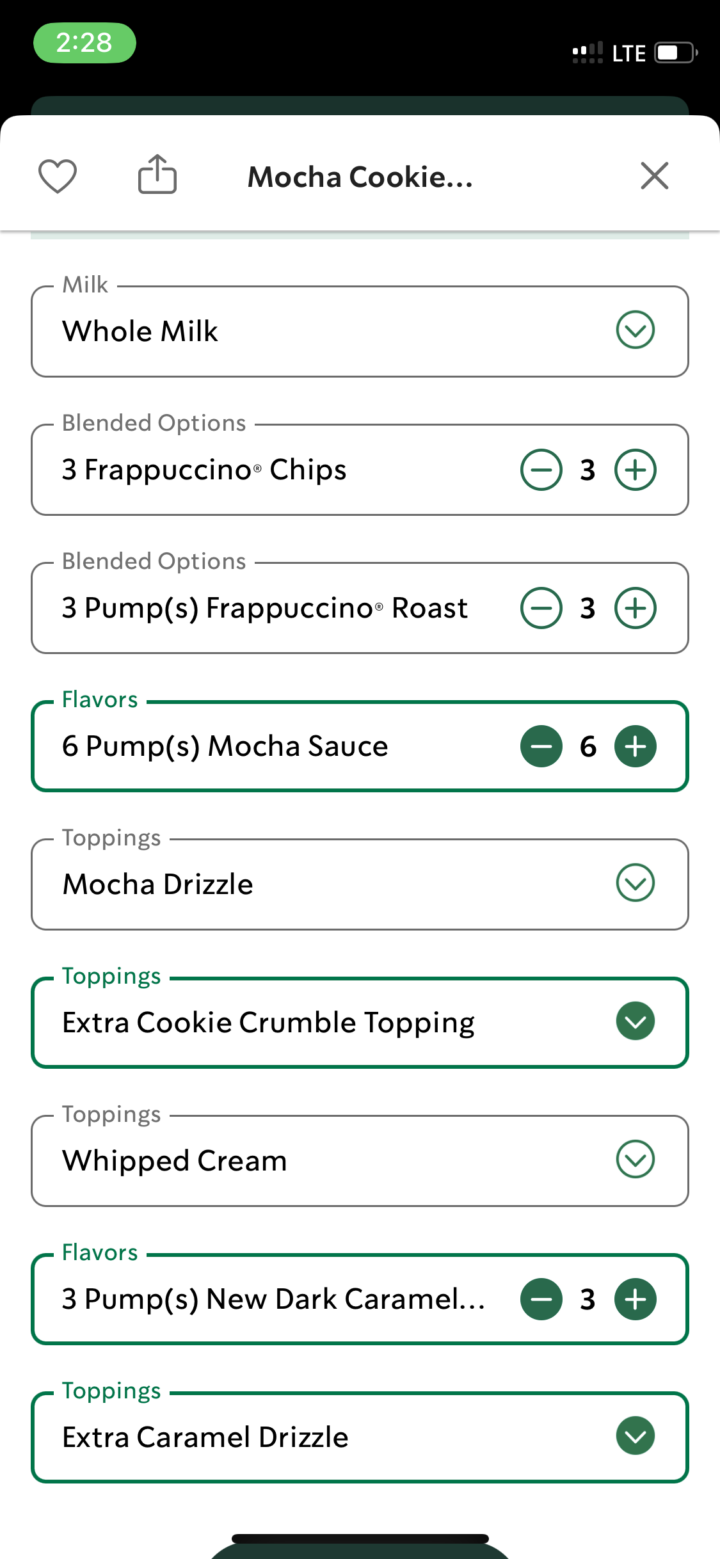The image showcases a detailed order page from a mobile device. The phone display indicates a mobile network connection with LTE and a battery level around half capacity. At the top of the screen, "Mocha Cookie" is prominently mentioned, suggesting the name of the drink being customized. The order shows a series of customizable options:

- **Milk:** Whole Milk
- **Add-ins:**
  - Three Frappuccino chips, adjustable via a plus-and-minus control.
  - Three pumps of Frappuccino roast, also adjustable.
- **Flavors:**
  - Six pumps of mocha sauce, with the plus-and-minus controls highlighted in dark green, indicating this selection is active.
- **Toppings:**
  - Mocha drizzle
  - Extra cookie crumbled topping, highlighted, implying this addition is selected.
  - Whipped cream
  - Three pumps of a new dark caramel sauce, highlighted and adjustable.
  - Extra caramel drizzle, suggesting a preference for extra caramel flavor.

Overall, the detailed order reflects a highly customized Mocha Cookie drink with multiple ingredient options and highlights specific selections in dark green for better clarity.